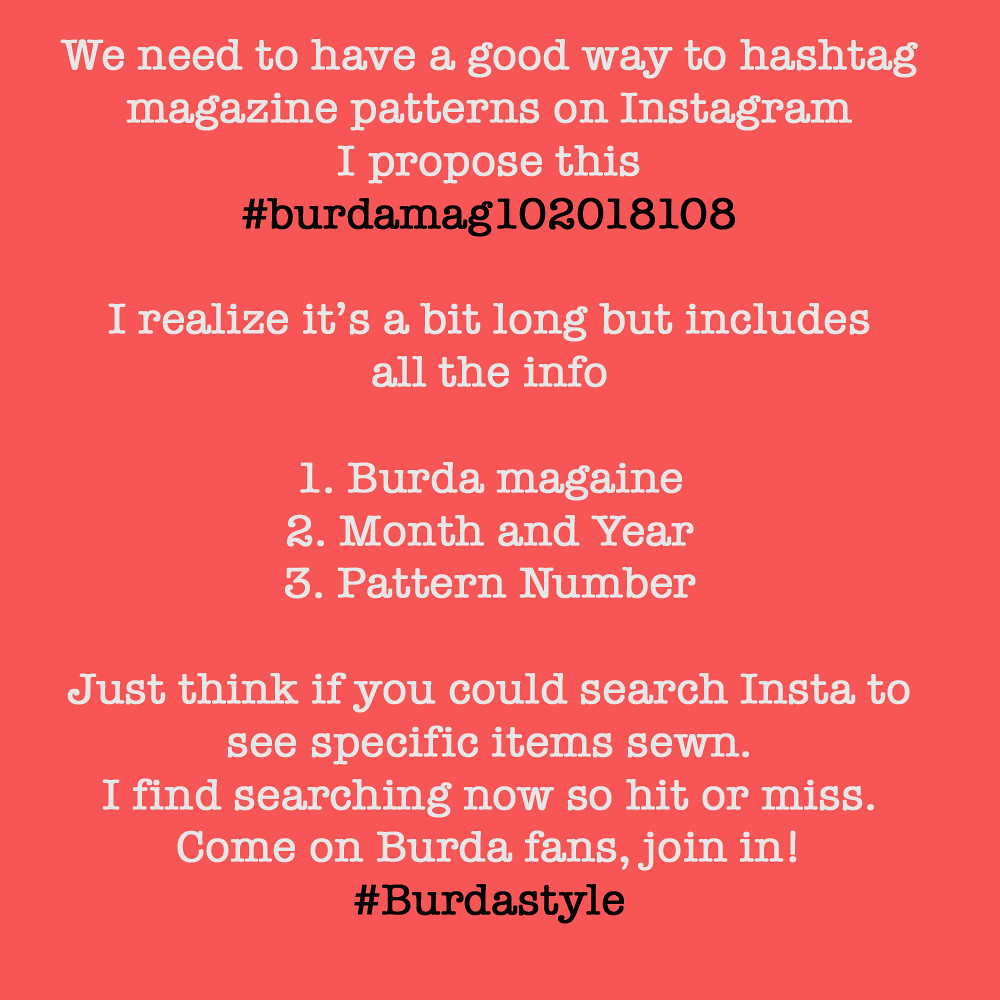This image appears to be an Instagram post focused on organizing and improving the searchability of magazine patterns using hashtags. The background is a bright melon or light red, leaning towards a salmon hue, with slight compression artifacts visible around the text. The text itself is predominantly in white, set in a simple typewriter-like font. At the very top, it states, "We need to have a good way to hashtag magazine patterns on Instagram," followed by a proposal for a specific hashtag.

The suggested hashtag, "#BurdaMag102018108," is prominently displayed in black font. Below this, the text continues in white, explaining, "I realize it's a bit long but includes all the info: 1. Burda magazine, 2. Month and year, 3. Pattern number." It emphasizes the utility of the hashtag for improving search functionality for specific items sewn, mentioning the current difficulties in searching patterns. The call-to-action encourages Burda fans to join in, ending with another hashtag, "#BurdaStyle," also in black font. Overall, the image is a clear, rallying call for a unified hashtag to better organize and search for sewing patterns on Instagram.